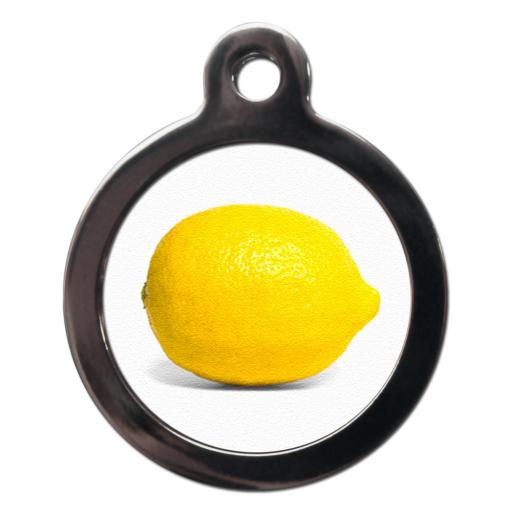The image features a whole, fresh, uncut lemon with a vibrant yellow peel, centered against a white background. The side view of the lemon reveals its textured surface, with the small stem end visible on the left and the peaked end noticeable on the right. Encircling this lemon is a thick black circular border, resembling a pendant or a magnifying glass frame. This black bezel has a small hole at the top, designed for hanging or threading a chain through. The simple yet striking composition is accentuated by the shadow of the lemon cast on the white background, making the bright fruit the focal point of the image.